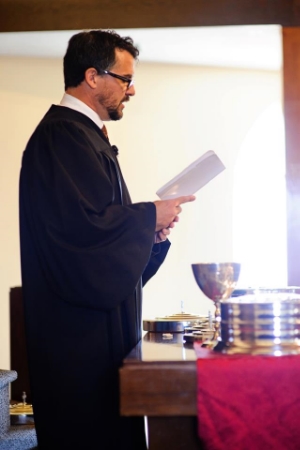In this image, a preacher is depicted in a solemn moment during a religious ceremony. He is wearing a black robe with voluminous sleeves and a white collared shirt underneath, possibly also donning a tie. The preacher, a white man with short black hair, a neatly trimmed black beard, and black-framed glasses, is engaged in reading from a folded white pamphlet he holds in his hands. A small microphone is affixed to his collar, indicating he might be delivering a sermon or leading a communion.

He stands beside a polished brown table adorned with a red cloth running across its center. On the table, there are several silver trays traditionally used for communion, with one large, deep chalice prominently placed in front of him. The table and its items appear to be ready for the sacrament, with the red cloth accentuating the solemnity of the occasion.

The scene is captured from a side view, with the preacher facing to the right. To the left of the table, there are gray carpeted steps, likely used for kneeling in prayer. The background is bright, with sunlight streaming into the room, creating glare and illuminating the white, or possibly off-white, wall which features a wooden border. The sunlit ambiance suggests it is daytime, adding a serene and reverent atmosphere to the image.